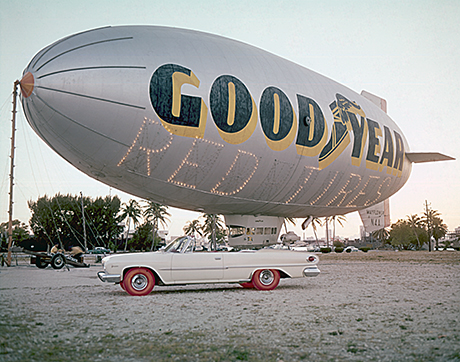A striking photograph captures a gray Goodyear blimp in the center, prominently featuring blue and yellow lettering spelling "Goodyear," with an iconic emblem and the phrase "RED TIRES" illuminated in dotted yellow, all in capital letters. Underneath the blimp, palm trees stretch across the scene. A white, classic convertible, showcasing red tires with silver rims, is positioned toward the left of the frame. The convertible is parked on a sandy terrain with patches of grass. In the background, the sky transitions from light blue to whitish, completing the picturesque setting.